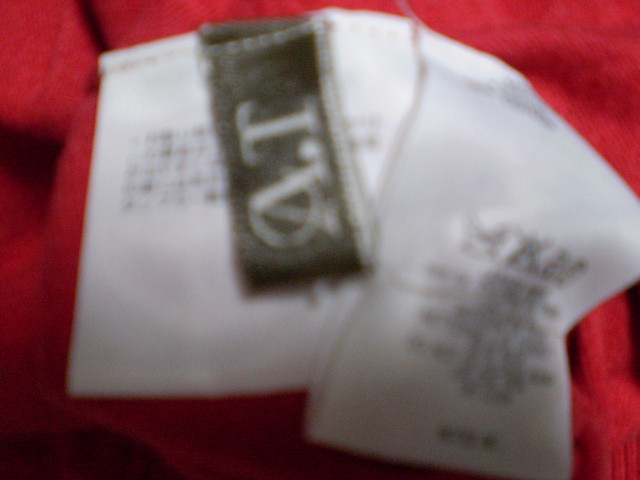This close-up photograph captures the back of a red sweater, though the image is entirely out of focus. Prominently displayed in the center are three tags. The largest tag is a white square, sewn directly into the sweater, featuring black text in its middle. Red stitching can be observed outlining the top of this tag. Overlapping this, a smaller vertical black tag is centrally positioned, bearing the letters "A.T." in bold white text. To the right of these, a third tag with machine washing instructions appears to have been detached and placed beside the other tags. The background reveals the knit texture of the red sweater, most noticeable in the bottom right corner of the photograph.